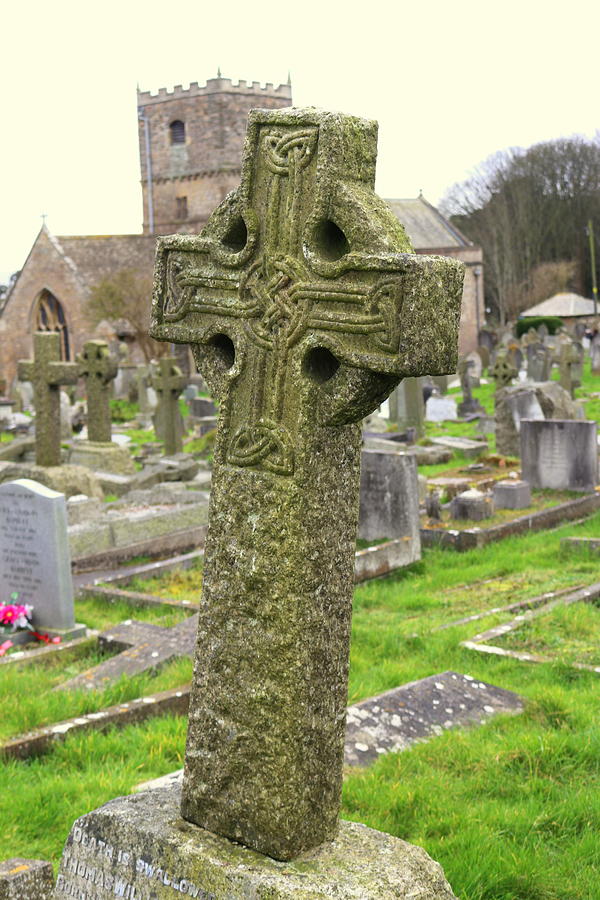The image depicts a serene outdoor cemetery with lush green grass spread across the area. Dominating the foreground is a prominent, weathered stone cross, heavily detailed with minor designs including lines and small leaf-like shapes at each end, and a crisscross pattern within a circle at its center. This large cross is firmly set into a rock pedestal, bearing an inscription partially readable as "death is something" and the name "Thomas."

Surrounding this central monument are numerous other tombstones, including several cross-shaped ones similar in style, particularly to the left of the main cross. Scattered red flowers adorn one of the rounded gravestones nearby, adding a touch of color to the scene.

In the backdrop, the view reveals a grand brick building that resembles a church or castle, complete with a tall tower featuring rectangular cutouts along its upper edge, reminiscent of a crown's battlements. The sky behind the building glows with a light pink hue, enhancing the tranquil atmosphere of the cemetery.